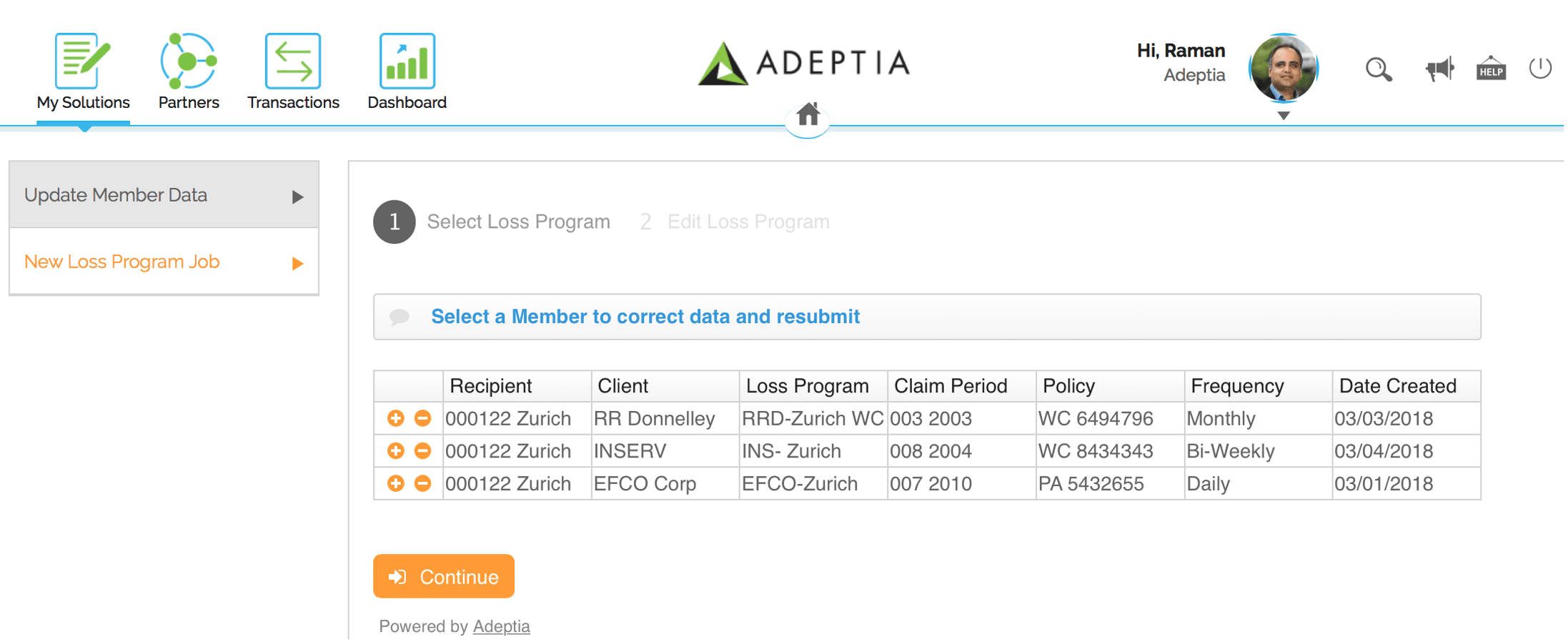The image features a clean white background with a section of blue and green icons at the top. The first icon, labeled "My Solutions" in black font with initial capitals, depicts a pen writing on a notepad. The second icon, labeled "Partners," resembles a steering wheel, while the third icon, labeled "Transactions," shows arrows pointing in opposite directions, indicating back and forth movement. The fourth icon, labeled "Dashboard," represents an ascending bar graph.

Central to the image is a logo featuring a triangle with an open, white triangular center. The outer portions of the triangle are colored green, matching the green used in the icons, and black. Above the triangle, the logo text "ADEPTIA" is displayed in all capital letters. 

To the right of the logo, the text "Hi Ramen" appears with "Adeptia" written underneath it in gray. Below this text is an icon depicting a bowl of ramen. Further to the right, a series of gray icons is lined up: a magnifying glass symbolizing a search function, a megaphone, a help icon, and a power button indicator.